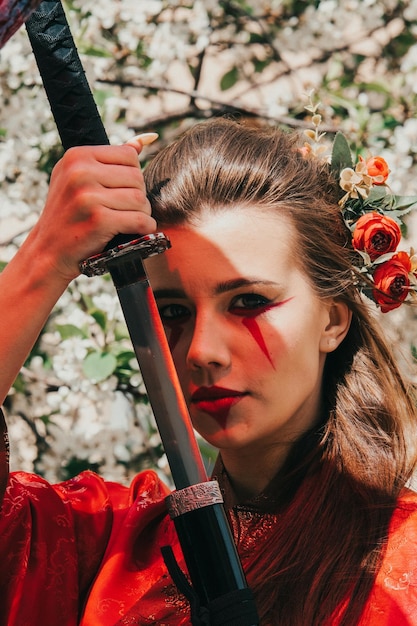The photograph portrays a young Caucasian woman in her late teens, depicted in a detailed and captivating cosplay attire. She dons a light red kimono, indicative of traditional Japanese attire, and accessorizes her medium-length brown hair with vibrant red and orange flowers. Her face is adorned with striking makeup; red lipstick, a downward red triangle beneath her lips, and red triangle accents extending from her eyes. Her complexion appears pale, enhancing the dramatic effect of her facial makeup. The woman holds a katana sword with her right hand, seemingly in the act of drawing the blade, with the bottom portion visible. She stands before a blossoming tree adorned with white flowers, adding a serene backdrop to the intense and focused expression on her face as she gazes directly at the viewer, exuding an aura of calm strength and beauty.